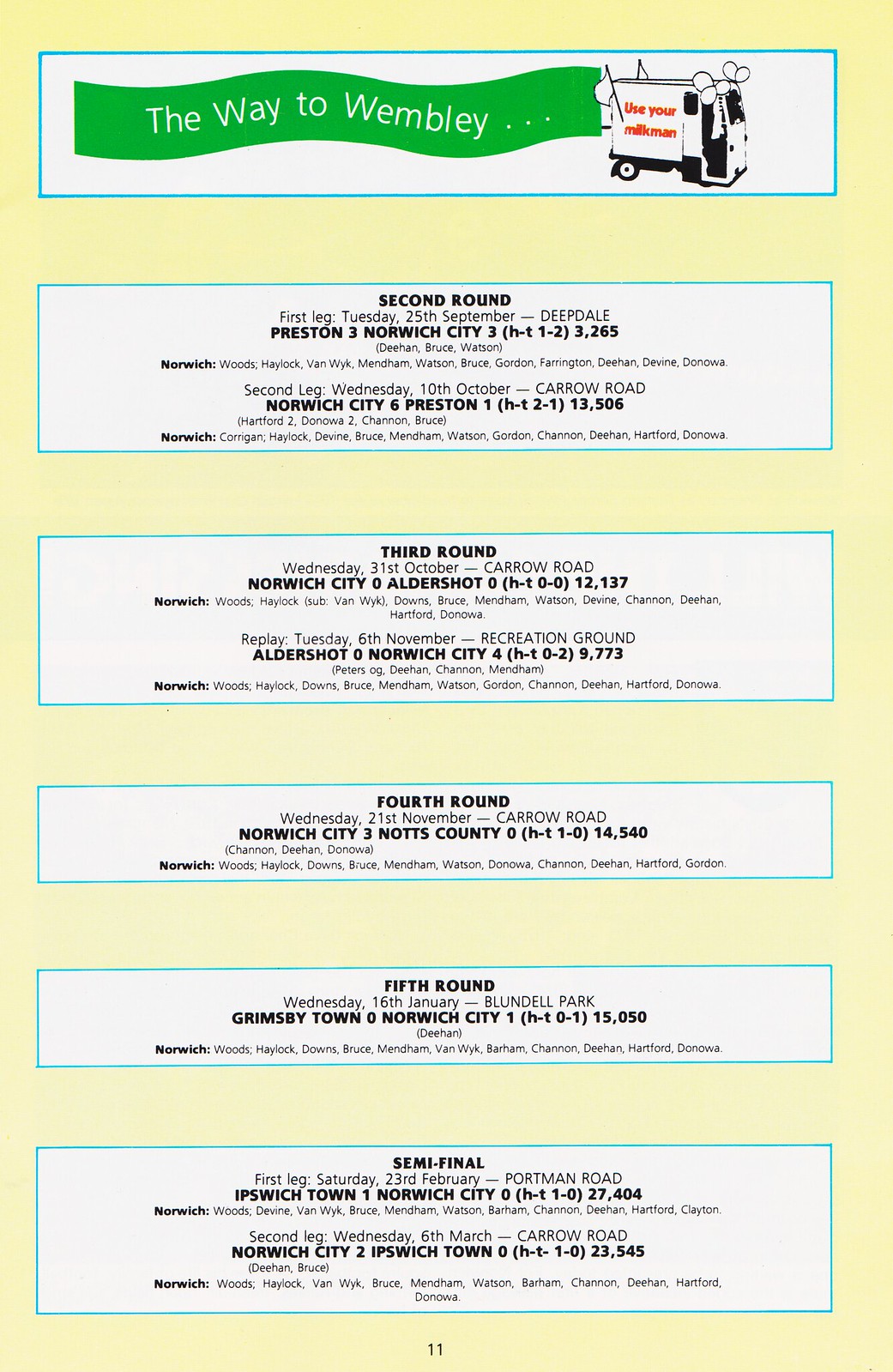This flyer, with a pale buttercream yellow background, is laid out in portrait orientation and features six horizontally arranged white rectangles outlined in a thin blue pinstripe. The top rectangle has a wavy green banner with white text stating "The Way to Wembley..." and, to its right, a whimsical drawing of a milk truck adorned with balloons and flags accompanied by the red text "Use Your Milkman." 

The subsequent rectangles document match details: 

- The second reads "Second Round, First Leg," listing the match on Tuesday, 25th September, between Deepdale, Preston (3), and Norwich City (3), with half-time scores and players' names, including Woods, Haylock, Van Wyk, Mendham, Watson, Bruce, Gordon, Farrington, Deehan, Devine, and Donowa. It also notes the second leg on Wednesday, 10th October, where Norwich City triumphed 6-1 over Preston.
 
- The third box outlines "Third Round" matches held on Wednesday, 31st October, resulting in a 0-0 draw between Norwich City and Aldershot. A replay on Tuesday, 6th November, saw Norwich City winning 4-0.

- The fourth box summarizes "Fourth Round" fixtures on Wednesday, 21st November, where Norwich City achieved a 3-0 victory over Notts County.

- The fifth rectangle details the "Fifth Round" match on Wednesday, 16th January, with Norwich City narrowly beating Grimsby Town 1-0.

- The final white rectangle covers the "Semi-final" stages: the first leg on Saturday, 23rd February, where Ipswich Town defeated Norwich City 1-0, and the second leg on Wednesday, 6th March, where Norwich City clinched a 2-0 win.

Overall, this page meticulously chronicles Norwich City's journey through various rounds of the tournament, highlighting key matches, dates, locations, scores, and players involved, all against a distinct yellow backdrop.